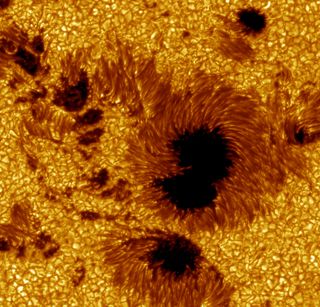The image is a highly zoomed-in, square close-up that captures an intricate and somewhat ambiguous subject—possibly the surface of the sun or the core of a flower. Dominated by vibrant yellow and orange hues, the background creates a bright, golden ambiance speckled with tiny light spots, giving a sense of texture and depth. Scattered across this radiant backdrop are 8 to 10 dark, black spots, each encircled by thick, reddish-brown, hair-like rays. These elements collectively evoke a sense of organic complexity, reminiscent of an artistic depiction or a detailed microscopic view. The image's detailed intricacies and the interplay of colors suggest an art piece or a magnified natural element, leaving its exact nature open to interpretation.